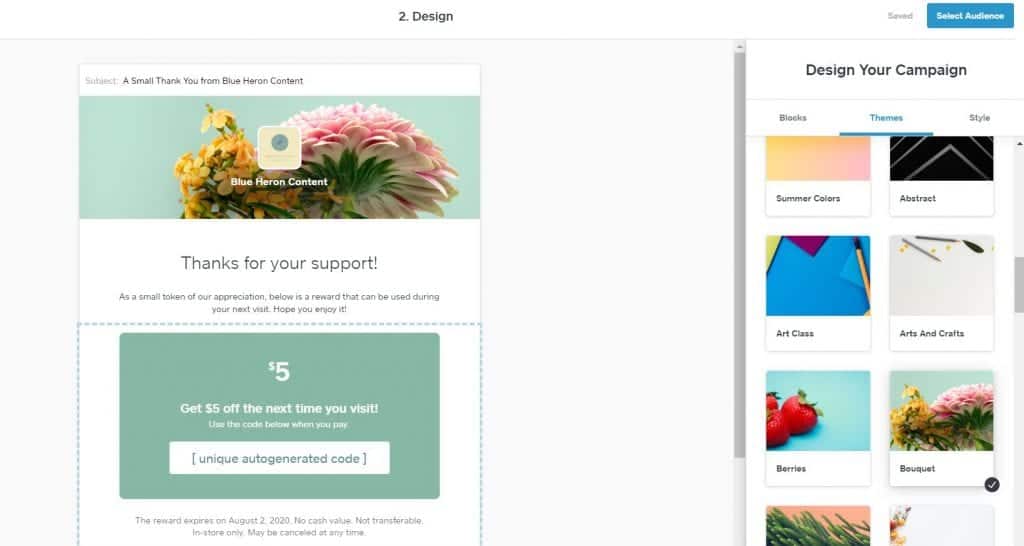The image showcases a close-up of a coupon page from Blue Heron Content. The page features prominently in the center, displaying a beautifully composed design with vibrant colors. At the top, elegant script reads "A Small Thank You from Blue Heron Content," setting a tone of gratitude. Beneath this heading, the design prominently features a stunning pink flower alongside a vibrant yellow flower, both set against a lush green background. The aesthetic is both inviting and serene.

A bold message in the foreground reads, "Thanks for your support. As a small token of our appreciation, below is a reward that can be used during your next visit. Hope you enjoy it." Directly under this message, a noticeable green box contains the text "$5," along with the offer details: "Get $5 off the next time you visit. Use the code below when you pay." The box includes a unique auto-generated code that can be clicked to reveal more details.

Important terms and conditions are also listed: "The reward expires on August 2, 2020. No cash value, not transferable, in-store only, may be canceled at any time."

To the right of the page, a section titled "Design Your Campaign" showcases different thematic categories such as "Summer Colors," "Abstract," "Art Class," "Arts and Crafts," "Berries," and "Bouquet." The text details provide a glimpse of the artistic options available, though it cuts off mid-description, leaving an element of curiosity.

Overall, the image effectively combines an expression of gratitude with visually pleasing elements and detailed information, inviting further interaction from the recipient.